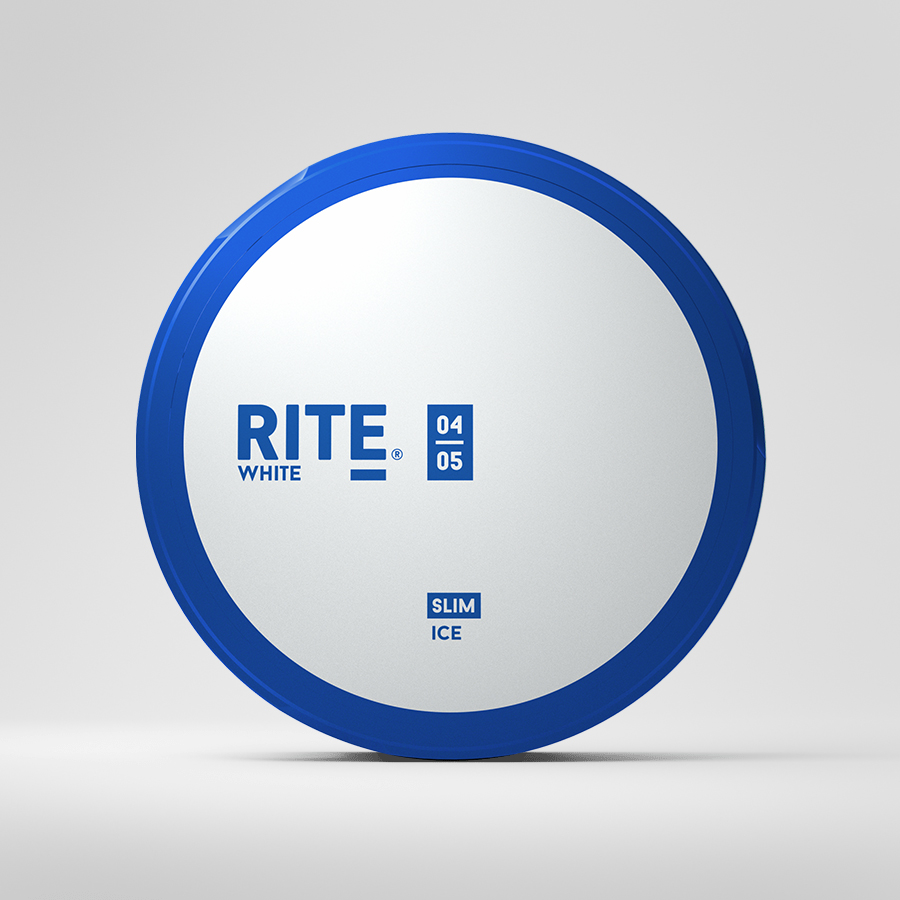The image depicts a circular product with a blue outer rim and a white center, set against a white background with a slight shadow beneath. The product is oriented so its flat side faces the camera. At the top center, in blue font, it has the text "RITE" with a registered trademark symbol by the "E". Below "RITE", the word "white" is written, where the "E" is underlined with a bold blue stroke. Adjacent to this text is a blue rectangular block containing the numbers "04/05" in white font, resembling a fraction. Towards the bottom of the disc, the word "SLIM" appears in white font within a blue color block, and the word "ICE" is in blue font on the white background. The entire object appears to be resting on an indistinguishable white surface that blends into the background.